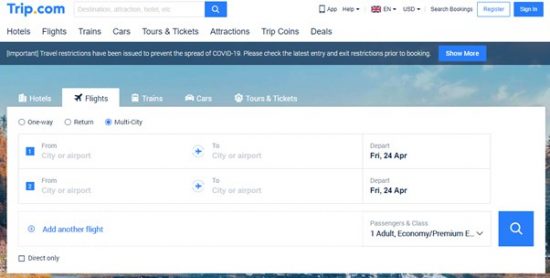A meticulously cropped screenshot of the top section of the Trip.com desktop website showcases a seamless and user-friendly interface. The header, pristine in white, prominently features the Trip.com logo emblazoned on the top left. Adjacent to the logo is a conveniently placed search box, facilitating easy navigation. Continuing to the right, the header includes essential links such as "App," "Help," a language and currency selection dropdown defaulted to "English, US Dollars," along with quick access to "Search Bookings," "Register," and "Sign In."

Beneath this structured header, the left-hand corner introduces a diverse array of travel categories: "Hotels," "Flights," "Trains," "Cars," "Tours & Tickets," "Attractions," "Trip Coins," and "Deals." These categories provide users with a comprehensive selection to tailor their travel experience.

Enveloping these features is a large, visually appealing photo that serves as a background, enhancing the overall aesthetic. Superimposed on this image are category buttons, with "Flights" being selected. This selection triggers a white dropdown box, partially obscuring the sky portion of the background photo.

Within the "Flights" section, users are presented with three travel options: "One-way," "Return," and "Multi-city," with "Multi-city" currently active. Below this selection, two input boxes prompt users to enter their departure ("From") and arrival ("To") cities, while the far-right box is designated for departure dates. A blue plus sign offers the functionality to "Add Another Flight." Adjacent to these features, the passengers and class dropdown box is preset to "One Adult, Economy Premium." A concise blue search icon, intuitively placed to the right, completes the search functionality, ensuring a streamlined booking process.

This detailed description captures the essence and functionality of the Trip.com website's interface, highlighting its intuitive design and user-centric features.